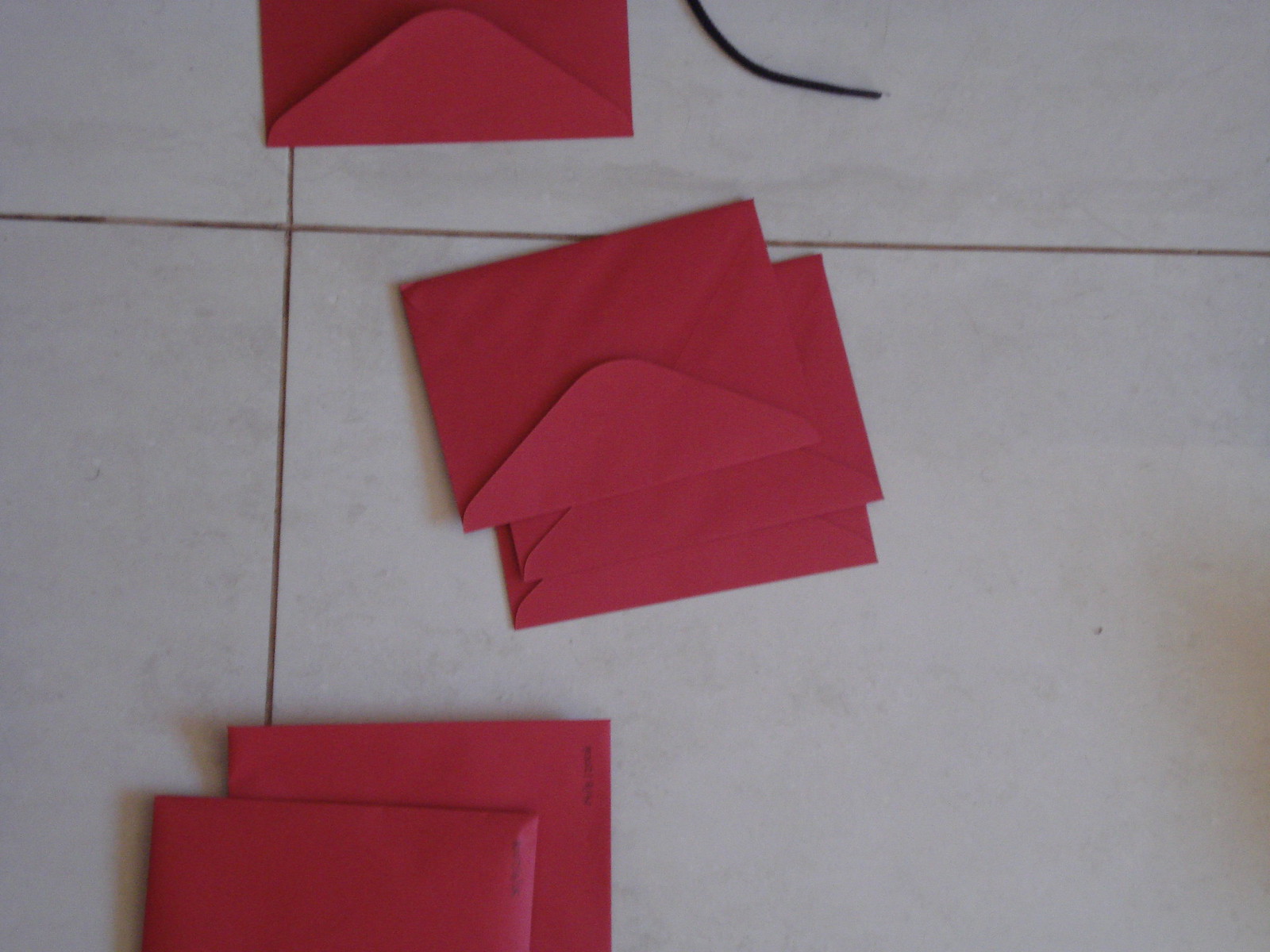The photograph captures a collection of six beet-red envelopes arranged on a medium grayish-green tile floor with narrow grout lines. The floor features large tiles, significantly bigger than those commonly used on countertops. At the top of the image, a black string or shoelace lies next to a single red envelope. In the center, there are three red envelopes positioned upside down, revealing their flaps. Towards the bottom, two more envelopes appear, slightly bulging as if filled, with black writing or a stamp partially visible on them. Shadows cast by the envelopes indicate varied lighting, adding depth to the composition. The overall scene suggests an indoor setting, possibly a kitchen or study area.